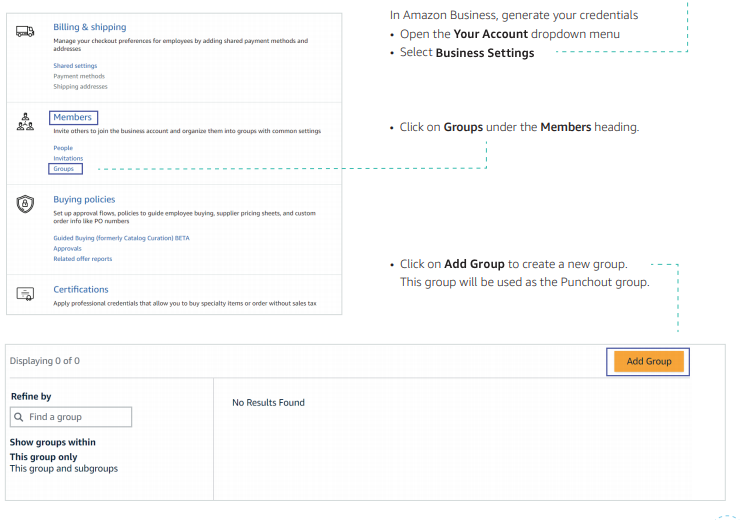The screenshot captures the configuration options for an Amazon Business account. The interface is clean, primarily white, with blue highlighted text and black text for content. The layout includes four distinct sections on the left side of the screen: "Billing and Shipping," "Members," "Buying Policies," and "Certifications." The "Members" section is currently highlighted, specifically under the subcategory "Groups."

The main page area features instructional text. The first line states, "An Amazon Business generates your credentials." Below this, there are two key options: "Open Account" and "Select Business Settings," with the latter being selected. Following this selection, the page directs the user to "click on 'Groups' under the 'Members' heading," indicated by a small arrow pointing to the highlighted "Groups" section.

Further guidance explains, "Click on 'Add Group' to create a new group. This group will be used as the punch-out group." Directly below, the section titled "Displaying 00" shows, indicating no groups have been added yet. The "Add Group" button is prominently highlighted in blue and orange for emphasis.

Finally, the bottom part of the page is allocated to fields for descriptor information on added groups. However, it currently displays "Displaying 0," confirming that no groups are present.